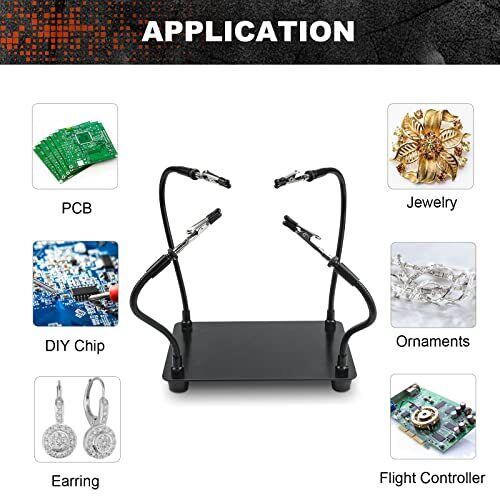The color image features a central object with a black rectangular base and four black wires extending from it, each ending in alligator clips arranged pointing towards the center. Across the top of the image, the word "Application" is prominently displayed. Surrounding the central object, there are six inset photographs grouped in pairs on either side. The left column's top photograph is labeled "PCB" and shows green computer chips. Below it, labeled "DIY Chip," is an image depicting a screwdriver manipulating some computer chip equipment. The bottom photograph in this column, labeled "Earring," shows a pair of silver earrings with clear stones. On the right column, the top photograph is labeled "Jewelry" and displays a gold leafy brooch. The middle photograph, labeled "Ornaments," features a detailed silver and glass object. At the bottom, labeled "Flight Controller," there is an image of a rectangular piece of hardware typically found inside a computer. The composition of the image suggests a diverse range of applications for the central device, from electronics and DIY projects to jewelry and decorative items.